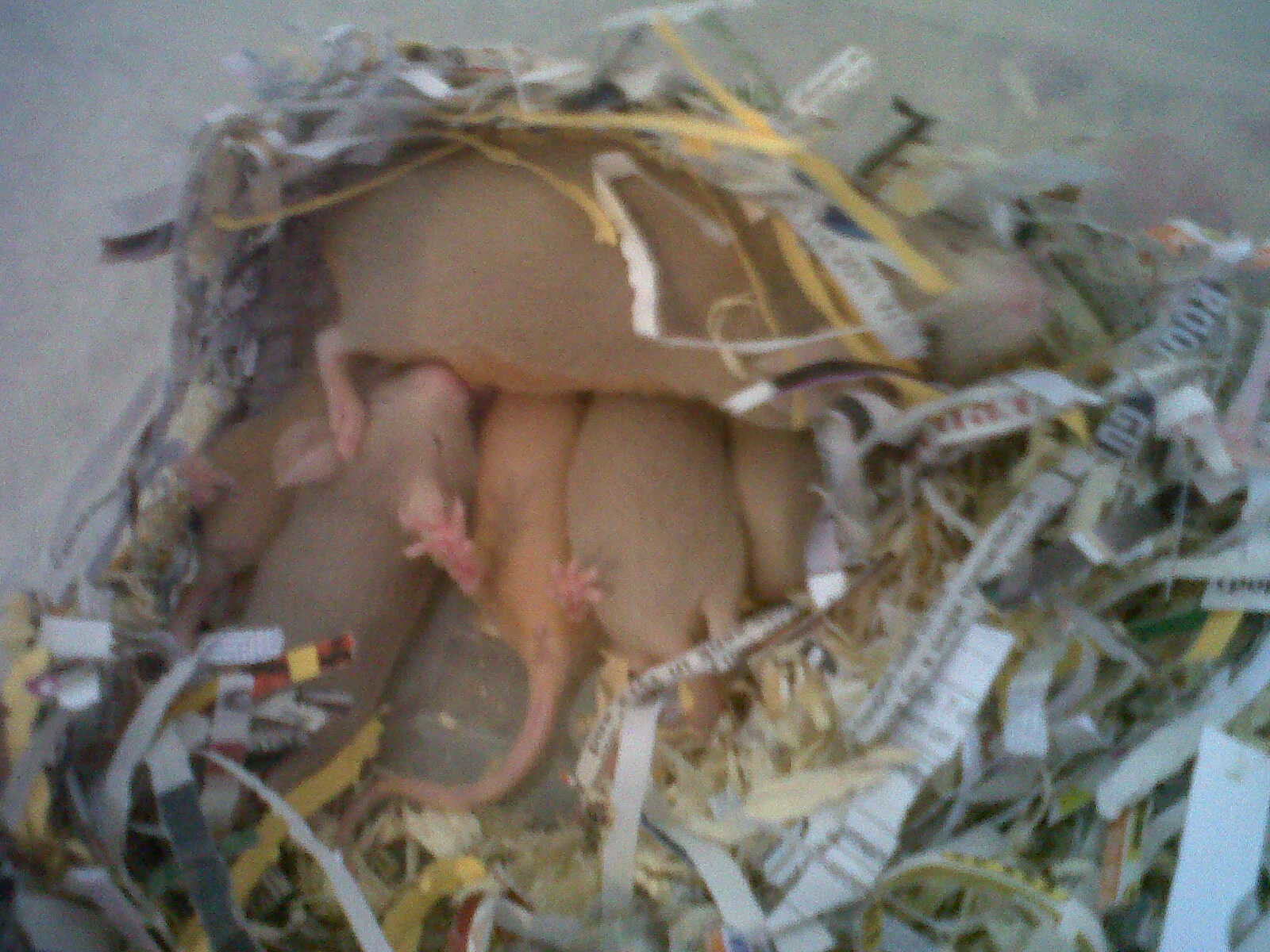An out-of-focus close-up captures a nest filled with what seems to be baby mice, nestled in a haphazard mix of shredded paper, straw, sticks, and labels. The background is a gray blur, which highlights the nest where six tiny mice are gathered, their light brownish-pink bodies just starting to grow fur. They have delicate pink feet and small tails. One of the mice is seen upside down, with its feet pointing skyward, apparently sleeping. The mice appear to be a week or two old, no longer newborn but still very young. It looks like a mother mouse may be present, feeding her babies beneath the shredded paper and nest materials, although it's somewhat hard to discern due to the blurry nature of the photo. The nest's construction from skinny strips of newspaper suggests that these mice might be raised in captivity.